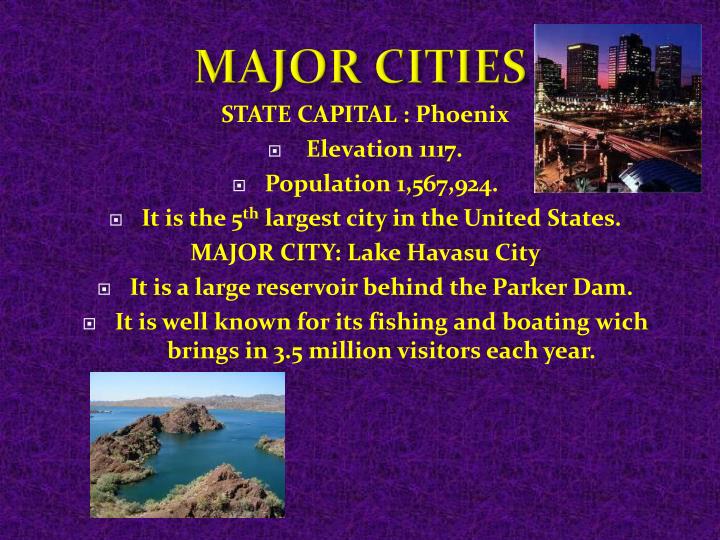The image features a predominantly purple and black background with a detailed overlay of yellow and white text. The text highlights key information about major cities in Arizona, prominently featuring the state capital, Phoenix, with an elevation of 1,117 feet and a population of 1,567,924, making it the fifth largest city in the United States. Another highlighted location is Lake Havasu City, known for being a large reservoir behind the Parker Dam, famous for its fishing and boating activities that attract 3.5 million visitors annually.

In the top right corner of the image, there's a vibrant cityscape shot of Phoenix at night, with the dark blue sky transitioning to a deep purple as if the sun is just setting. The scene includes illuminated buildings and motion-blurred traffic, suggesting a lively urban environment. The bottom left corner displays an aerial view of Lake Havasu, showing clear blue waters surrounded by green and brown mountainous terrain, interspersed with vegetation-filled land areas, encapsulating the lake's desert surroundings.